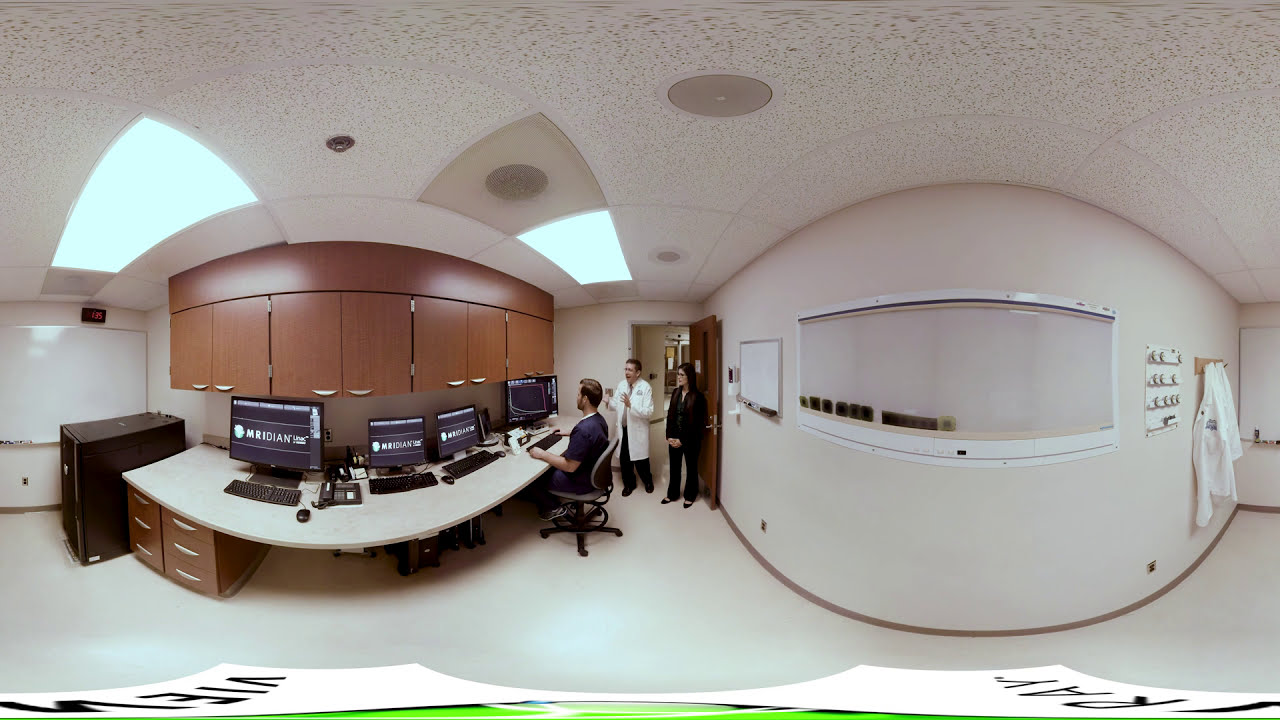The photograph depicts a bustling, white-walled doctor's office equipped with several black computer monitors and accompanying keyboards, all arranged neatly on a white desk. The office is bathed in bright, fluorescent light emanating from the ceiling, dotted with silver water sprinklers and gray speakers. The setting also includes brown cabinets and drawers, a black file cabinet, and multiple white dry erase boards with visible text such as "RAY" and "VIEW" written in black letters. 

In the room, there's a seated technician in blue scrubs working at the computer station, with black mouses and phones scattered about. To his left stands a doctor dressed in a white lab coat and black pants, while a woman in an all-black outfit stands nearby. The background includes a prominently brown door, a window, and white doctor's coats hanging up on the walls, which appear somewhat curved, accentuating the room's circular design. The floor is also white, completing the clean and sterile environment indicative of a medical facility geared toward diagnostics and patient care.